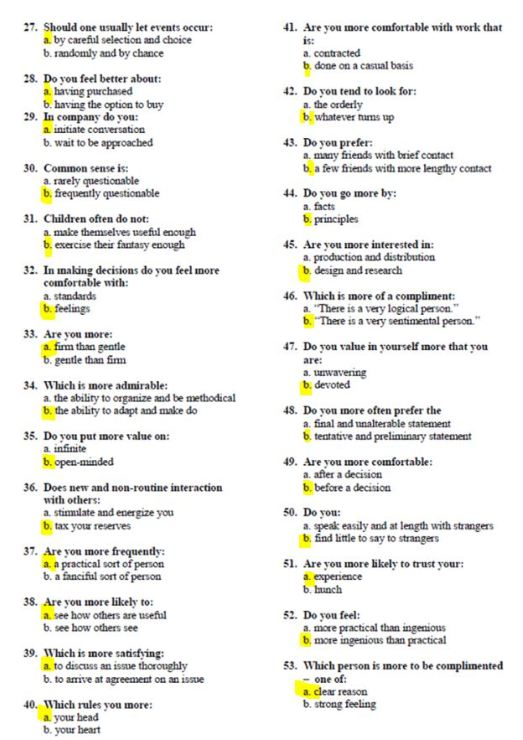The image features a white background with two columns of numbered questions, each containing two answer options. The left column ranges from numbers 27 through 40, while the right column ranges from numbers 41 through 53. Each question has one of its answer options highlighted in yellow, indicating the correct response according to the depicted quiz or test.

For example:
- Question 27 reads, "Should one normally let events occur (A) by careful selection and choice, or (B) suddenly and/or randomly and by chance?" Option A is highlighted in yellow.
- Question 24 queries, "Do you feel better about (A) having purchased or (B) having the option to buy?" Both options A and B are highlighted.
- Another question states, "Common sense is (A) really questionable or (B) frequently questionable," with option B highlighted in yellow.

The font used appears quite small, posing difficulty in reading the text when trying to zoom in.